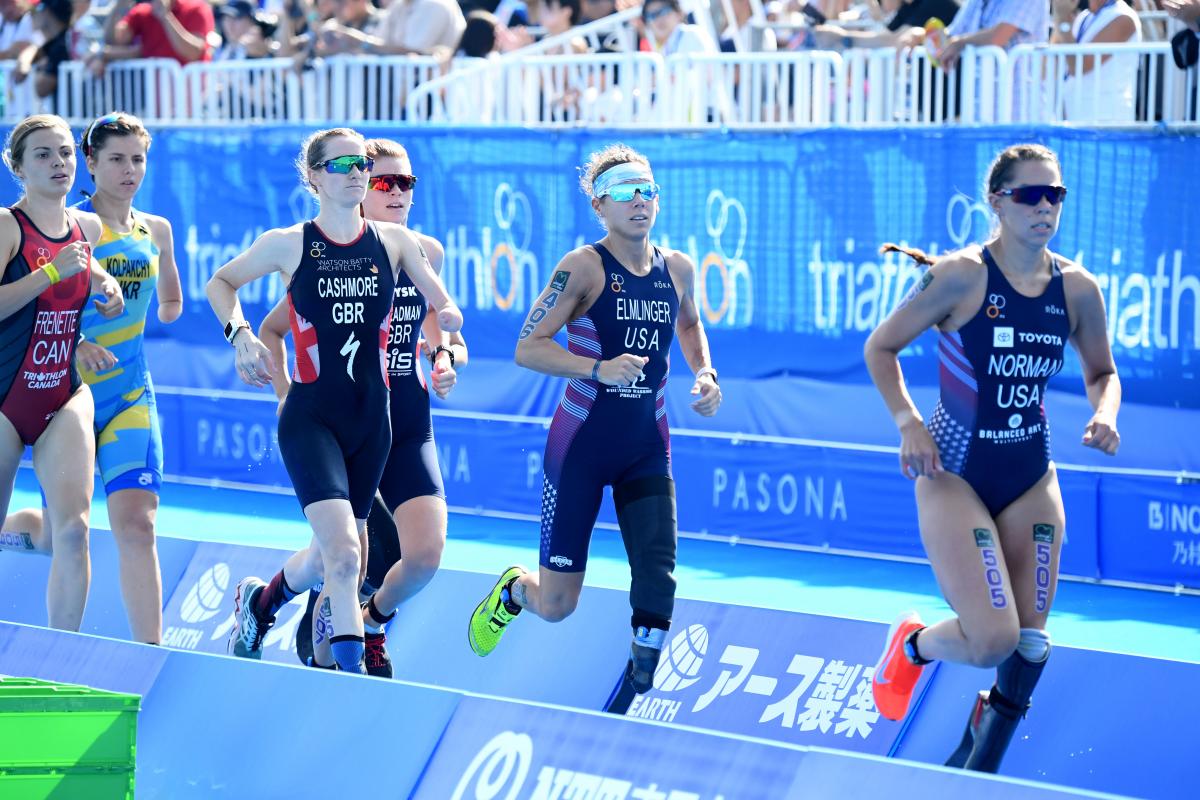This is a detailed photograph of a women's race, potentially part of a Paralympic triathlon given the presence of athletes with prosthetic limbs. In the image, six women are competing on a track flanked by triangular barriers. The leading athlete, identified as Norman from the USA, wears a Toyota-sponsored jersey, red or orange Nike sneakers, and has a prosthetic on her left leg. She features brown hair tied in a long braid and sports sunglasses. The second-place runner is also from the USA and has a prosthetic leg. The participants represent various countries displayed on their uniforms, including the USA, Great Britain, and Canada. A prominent blue banner in the background reads "triathlon" along with Olympic rings, suggesting an official triathlon event. Behind the blue backdrop is a white metallic partition with spectators barely visible at the top of the photograph, attentively watching the race.